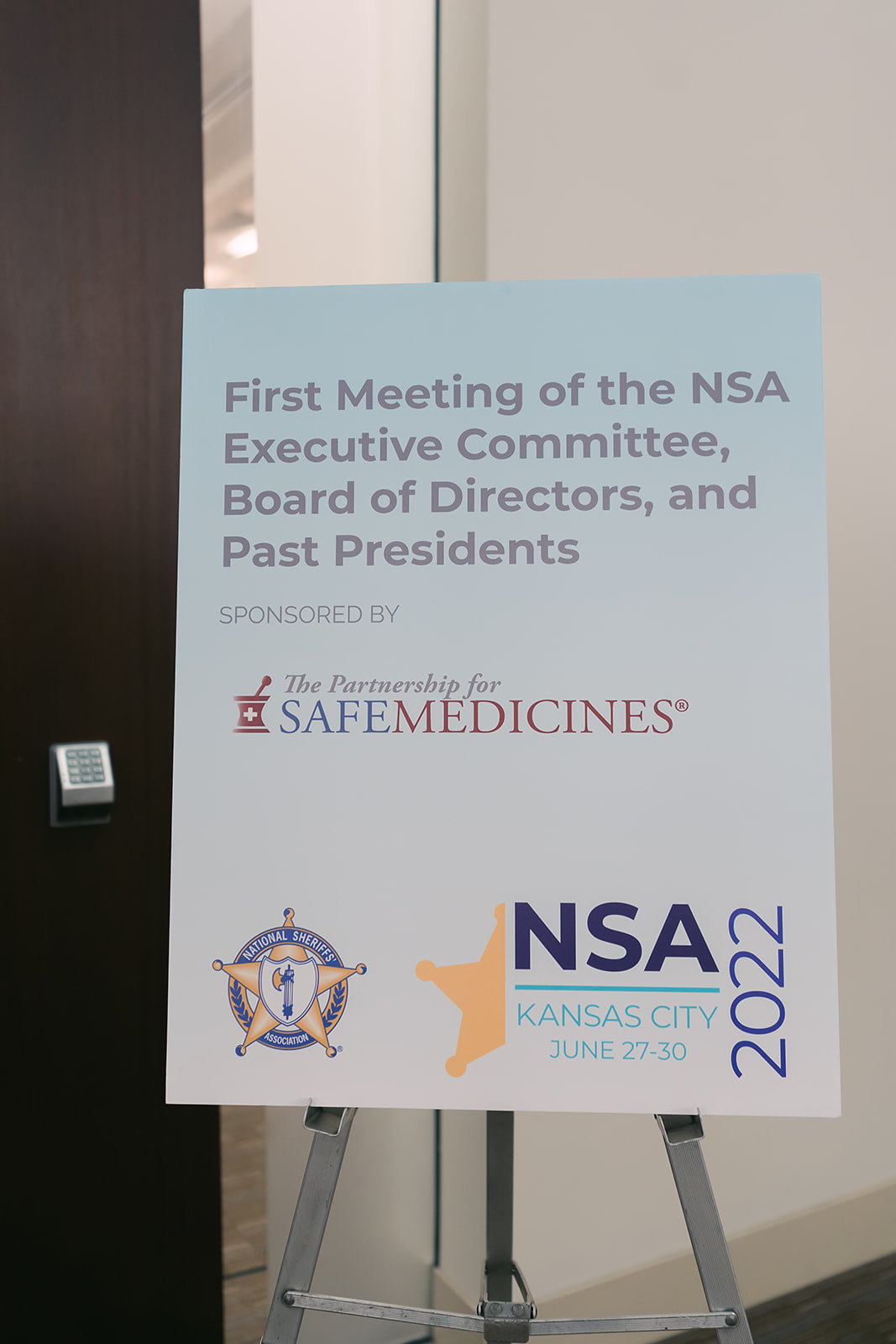The photograph showcases an indoor setting dominated by a large white cardboard sign mounted on a metal tripod. The sign prominently announces, in gray font, the "First Meeting of the NSA Executive Committee, Board of Directors and Past Presidents, sponsored by the Partnership for Safe Medicines." To the left of this text is a red mortar and pestle logo, featuring a plus sign. In the lower right-hand corner, the text reads "NSA Kansas City, June 27-30, 2022," accompanied by a graphic of half a yellow sheriff's star. In the lower left-hand corner, the full logo of the National Sheriffs Association is displayed, consisting of a yellow sheriff's star encircled by blue text and featuring a shield with an axe in the center. The background includes a white wall, a white door with a doorway to its left, and a partially open tall brown door with a keypad entry system. The overall setting indicates a professional event location, possibly a convention hallway.